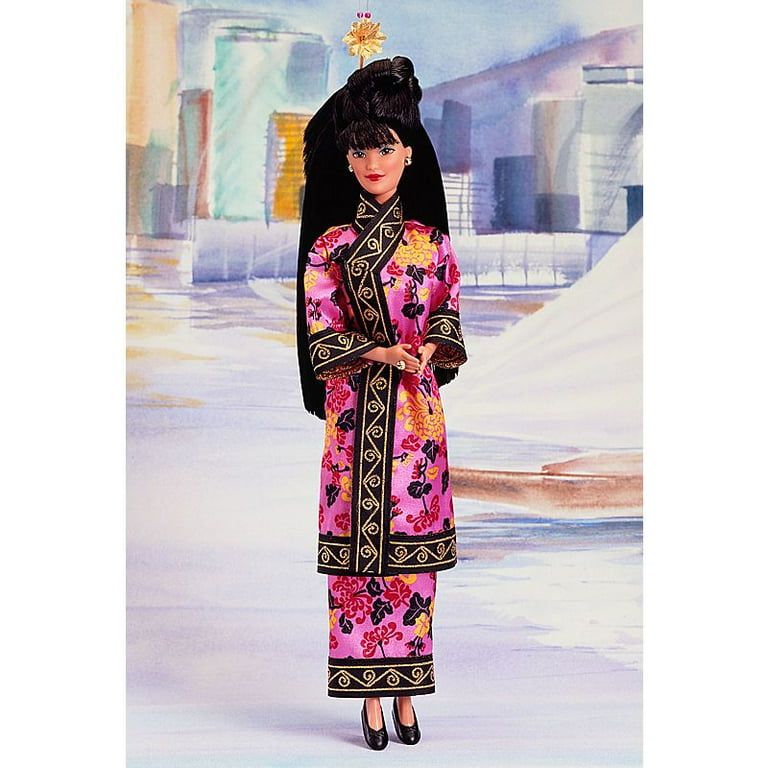In this composite image, a custom-made Asian-style Barbie doll is prominently featured against a watercolor backdrop depicting a modern cityscape with minimalistic skyscrapers suggested by simple rectangle shapes and sparse window lines. The Barbie doll, posing on what resembles a concrete slab, showcases a stunning pink kimono adorned with gold trim and floral patterns in yellow, red, and black. She wears black high heels, long black hair with bangs, and accessorizes with solid earrings, a ring on her right ring finger, and blue eyeshadow complementing her brown eyes and red lipstick. The image combines the physical realism of the doll with an artistic city background, creating a vivid contrast between the detailed figure and the abstract urban scenery.